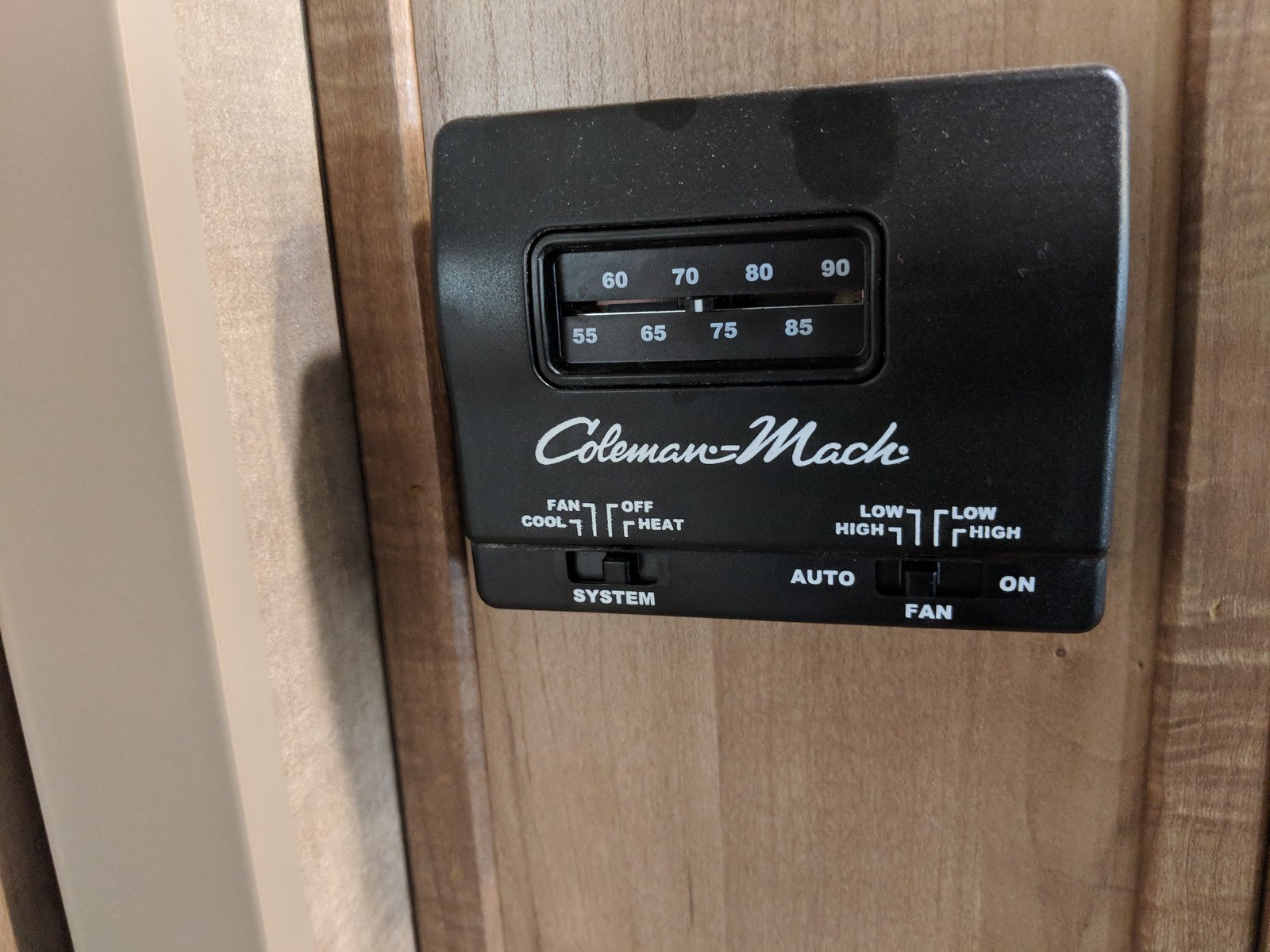This close-up photograph showcases a classic, dust-covered thermostat mounted on a vertical wall adorned with brown paneling. The thermostat is positioned in the upper right quadrant of the image. The brown paneling on the wall contrasts with a lighter brown doorway that edges into the frame on the far left side. The thermostat itself, a rectangular device oriented horizontally, is black and features white text, indicative of a basic model. It reads temperatures from 55 to 90 degrees Fahrenheit with a prominent temperature indicator line. Brand markings "Coleman Mac" are visible beneath the temperature scale. The device has two switch panels; the left switch is labelled with "system" functions including cool, fan, off, and heat. The right switch controls the fan settings marked as "auto" and "on," and includes speed options "low" and "high." Evident on the thermostat are fingerprints and dust, adding an element of everyday use and age.